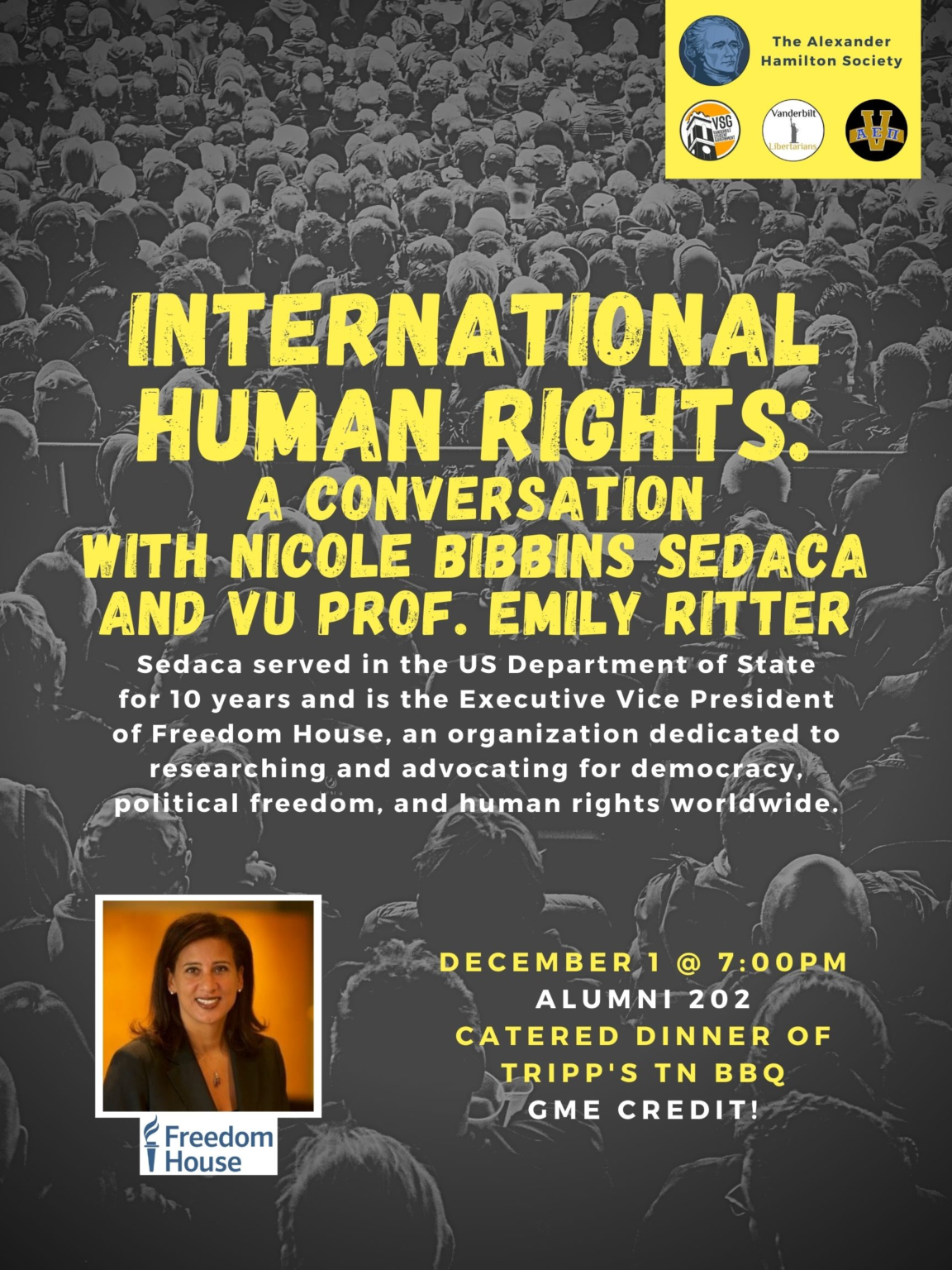The flyer promotes an event hosted by The Alexander Hamilton Society, featuring an in-depth conversation on international human rights. The background depicts a theater audience viewed from behind in varying shades of light and dark gray.

In the top right corner, the flyer displays the Alexander Hamilton Society logo, with three smaller circles containing illegible text beneath it. 

The main event details are prominently centered in yellow text: "International Human Rights: A Conversation with Nicole Bibbins Sadaqa and VU Prof Emily Ritter." Below this, a white text blurb provides background information on Nicole Bibbins Sadaqa, noting her ten years of service in the US Department of State and her current role as Executive Vice President of Freedom House, a leading organization devoted to promoting democracy, political freedom, and human rights worldwide.

An image of a woman with brown hair wearing a suit jacket, identified as being from Freedom House, sits in the bottom left corner against a burnt orange background.

Further event details are in yellow and white text to her right: "December 1st at 7 p.m., Alumni 202, Catered Dinner of Trips, TN BBQ, GME Credit." Notably, "Alumni 202" and "GME Credit" are highlighted in white, while the remaining details are emphasized in yellow and fully capitalized.